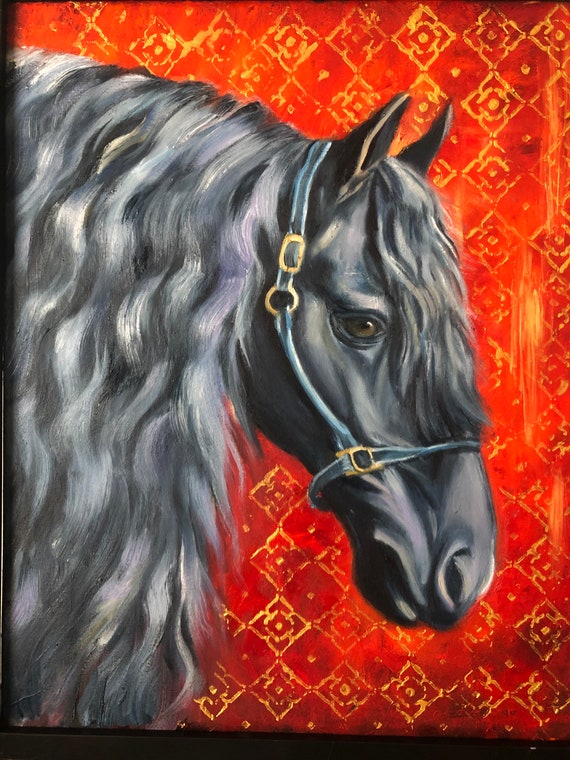This detailed painting, possibly computer-generated, portrays a serene black Frisian horse with an exquisitely long, wavy white mane cascading to the right side of its neck and a forelock draping between its deep brown eyes. The horse's limpid eye faces the viewer, conveying a gentle, perhaps slightly forlorn expression. Adorned with a blue bridle featuring gold accents, the horse stands against a luxurious red background decorated with gold diamonds, each containing a floral motif. The intricately rendered horse, seemingly only visible from the neck down, contrasts beautifully against the brocade-inspired backdrop, showcasing a high level of artistry and finesse.